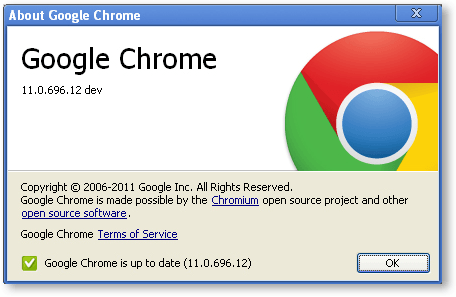Here is a cleaned-up and detailed caption for the described image:

---

The page features an interface outline in a medium blue color at the top left corner. At the very top, displayed in a basic sans-serif white font with noticeable letter spacing, there is the text "About Google Chrome." The font appears slightly fuzzy as if the image quality is low. The blue bar at the top is significantly thicker compared to the side and bottom borders.

Below this, there is a white background with a prominent large, bold black font stating "Google Chrome." Beneath the main header, in a more digitized and lowercase font, the version number "11.0.696.12 dev" is indicated.

Towards the right, about two-thirds of the Chrome logo is visible. The logo is a circular design with a central blue circle outlined in white, and the remaining segments are colored green, red, and yellow.

At the bottom of the page, there is a section in a beige color reminiscent of traditional Windows 98 to Vista notification themes. This section includes the text, “Copyright © 2006 to 2011 Google Inc. All rights reserved.” On the next line, it states, "Google Chrome is made possible by the Chromium," with the word "Chromium" underlined in blue to indicate a clickable link, followed by "open source project and other open source software." Here, "open source software" is also underlined in blue to denote a clickable link.

Further down, the text "Google Chrome Terms of Service" appears twice, each instance underlined in blue, indicating clickable links that likely redirect to another window.

In the bottom section, there is a green box with a white checkmark and the text "Google Chrome is up-to-date (11.0.696.12)." To the right, there is an "OK" button within a rounded rectangle, which has a dotted interior border and an outer blue border.

---